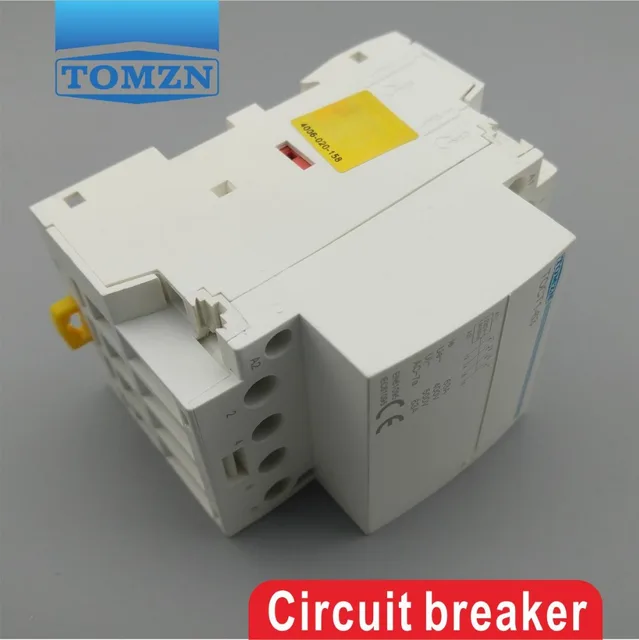The image is a color photograph featuring a white plastic circuit breaker prominently placed against a plain gray background. In the top left corner, the company name "T-O-M-Z-I-E-N" is displayed in blue letters. On the circuit breaker's top surface, there is a yellow sticker that appears to have the number "4006-020-158." The circuit breaker includes an orange or yellow plastic hook at its bottom, as well as several round holes. On the side of the circuit breaker, a vertical blue stripe is positioned above the letters "T-O-C-T," followed by a column of gray text that likely contains technical details such as dimensions or voltage information. In the bottom right corner of the image, a red rectangular label with white lettering indicates the product is a "Circuit Breaker."